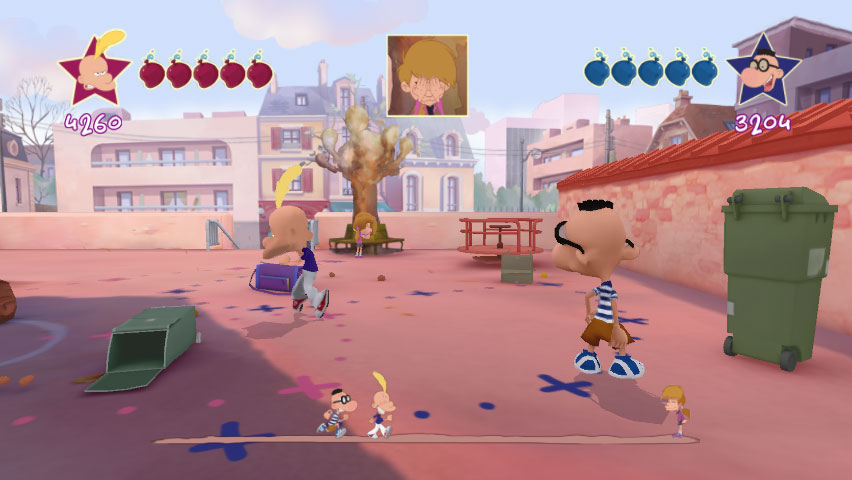The image depicts a vibrant scene from a game featuring two animated characters engaged in competition. On the top left corner, there is an emblem of a purple star alongside five purple apples, with a score of 4260 displayed below. This side is represented by a character with an animated, blond-haired child at the center. On the top right corner, a blue star emblem with a smiling face wearing glasses is shown, accompanied by five blue apples to its left and a score of 3204 underneath. This right-hand character is dressed in blue and white sandals, brown shorts, and a blue and white shirt, while the left-hand character wears white pants and a blue shirt.

The setting is a mostly pink ground base adorned with numerous pink and blue dots and Xs. There is a knocked-over green container situated centrally in the image. To the right, a second green dumpster is visible, adjacent to the edge of a building with a pink facade and a red rooftop. The background showcases a series of buildings surrounding a boxed-in courtyard, completing the lively game environment.